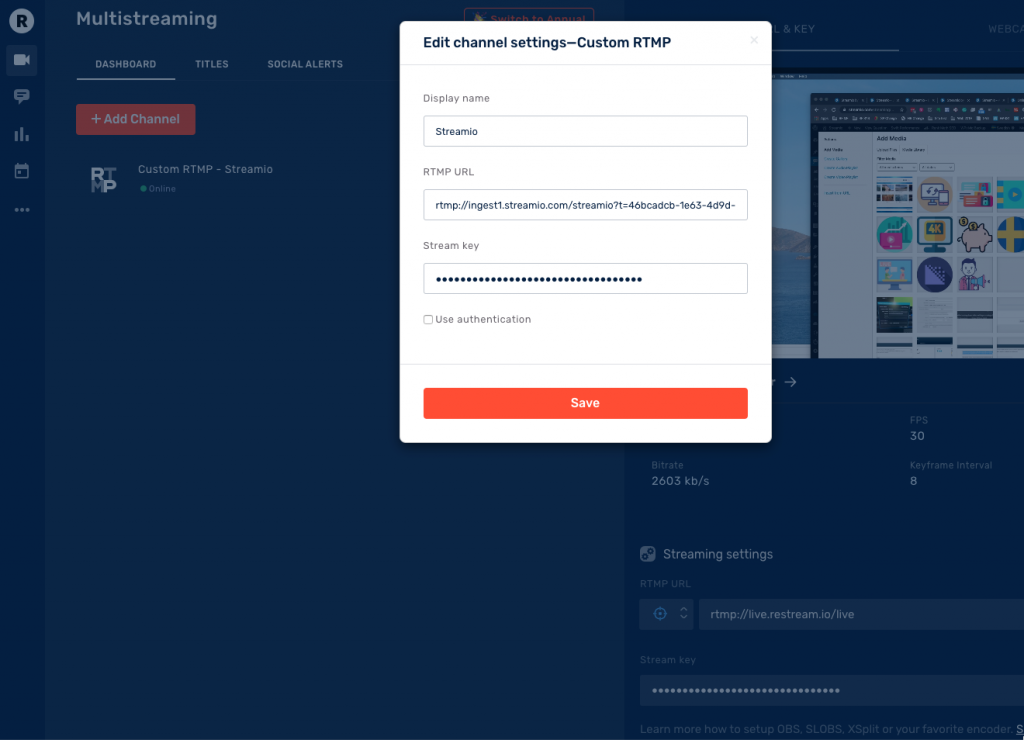**Caption:**
The image depicts a webpage interface under the category of streaming websites, featuring a predominantly blue background. In the upper right-hand corner, icons for various functions are present: an 'R' icon, a video camera, and a messaging icon, signifying available features. Adjacent to these icons, in the next column, is the multi-streaming option, which is highlighted due to the video camera icon being active.

The interface displays a menu with options such as "Dashboard," "Titles," and "Social Alerts," with the "Dashboard" currently highlighted. Beneath the main menu, there are selections for "Add Channel" and "RTMP custom RTMP streams." A pop-up window on the screen shows "Edit Channel Settings" for a custom RTMP stream. The fields within this pop-up include a "Display Name" field, populated with "Streamio," and "RTMP URL" and "Stream Key" fields, the latter represented by obscured dots for privacy. There’s also a checkbox labeled "Use Authentication," and buttons for "Save" and "Cancel."

To the right of the pop-up, there is another blue box titled "Streaming Settings," which lists details like "RTMP Live" and "restream.io.live," followed by another hidden password. The detailed elements of the interface suggest that the site is a comprehensive streaming service platform.